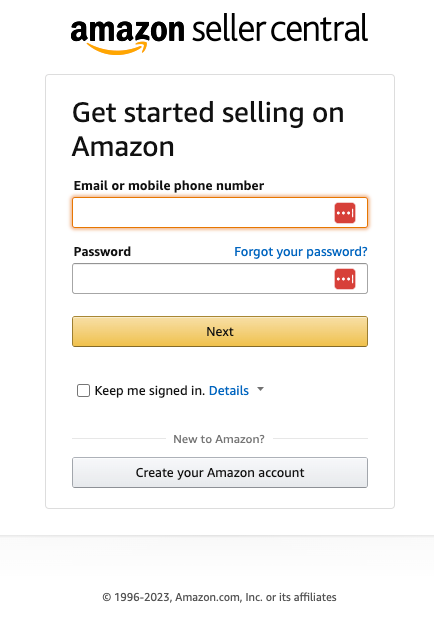The image is a screenshot of the Amazon Seller Central login page, featuring a clean, all-white background. At the top, the header clearly displays "Amazon Seller Central" alongside the Amazon site arrow. Beneath this header, there is a central white box with the message, "Get Started Selling on Amazon."

Following this, users are prompted to enter their email or mobile phone number into a designated input field. Below that, there is a field for the password with a clickable blue text saying, "Forgot Your Password." Further down, a prominent yellow rectangle button labeled "Next" stands out.

Additionally, there is an option labeled "Keep Me Signed In" with a clickable checkbox next to it. Near the bottom of the screen, a message reads, "New to Amazon?" beside a gray button that encourages users to "Create Your Amazon Account."